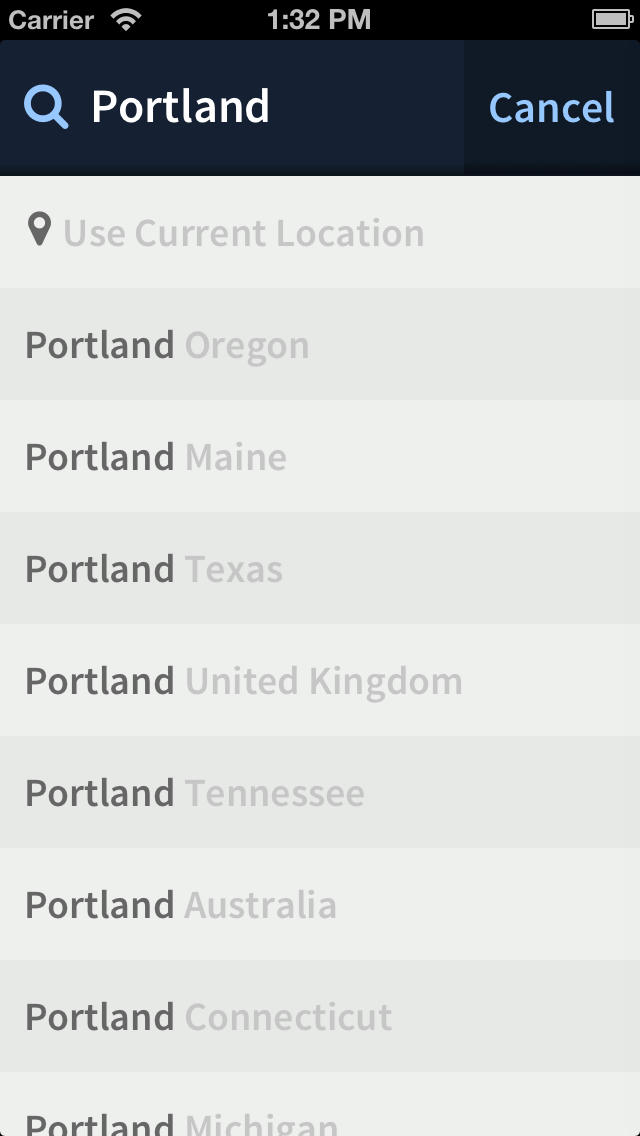This is a detailed screenshot depicting a mobile phone interface. 

At the very top, there's a status bar with various indicators on a solid black background. On the far left, the word "Carrier" is displayed alongside a full-strength Wi-Fi signal icon. Adjacent to this, the current time is shown in gray text, indicating "1:32 p.m." On the right side of the status bar, a full battery icon is also visible.

Beneath this status bar, there is a search bar with a blue magnifying glass icon on the left and the word "Portland" typed into the text box. To the right of the text box, the word "Cancel" appears in blue.

The background below the search bar features a pattern alternating between gray and dark gray. Immediately below the word "Portland" in the search bar, a light gray option reads "Use current location," accompanied by a dark gray location symbol.

Below this, there are four search results for "Portland" each with a dark gray title followed by a light gray subtext indicating the region:
1. "Portland" with "Oregon" beneath it.
2. "Portland" with "Maine" beneath it.
3. "Portland" with "Texas" beneath it.
4. "Portland" with "United Kingdom" beneath it.